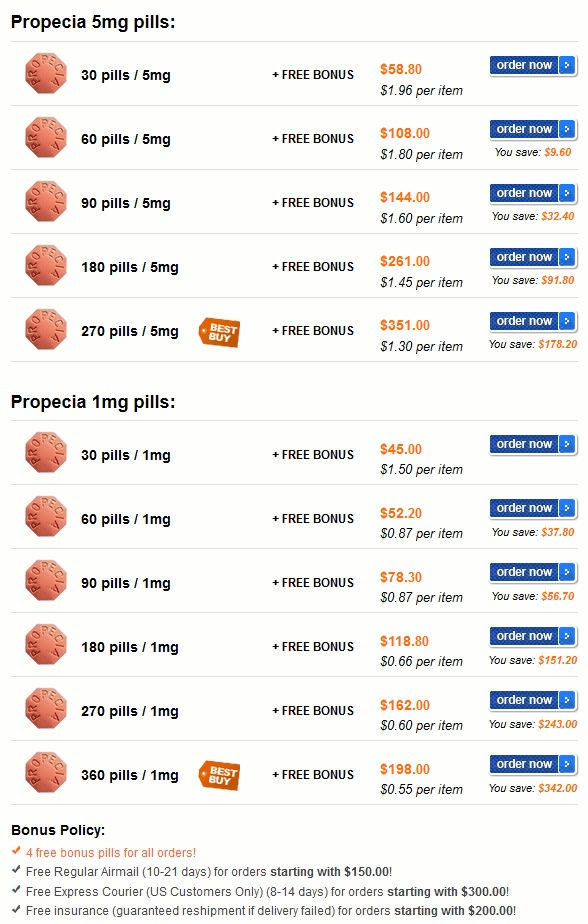The image appears to be a screenshot from an online pharmacy website, specifically showcasing an order page for the medication Propecia. At the top left corner, there is a listing for 5 milligram Propecia pills. The pill is described as octagonal in shape and has a rosy red, almost peach color, with the name "Propecia" printed along its edges.

Beneath this listing, small images of the pill are displayed. In the adjacent column, various purchasing options for the 5 milligram pills are shown, starting from quantities of 30 and scaling up to 60, 90, 180, and 270. Further down, there's a category for the 1 milligram Propecia pills, which also come in multiple quantities that seemingly increase by intervals of 30 or 60.

To the right of these selections, free bonus offers are highlighted in black text, and next to these, the prices are listed. The 5 milligram pills start at $58.80, while the 1 milligram pills are priced from $45. Each row corresponding to a different quantity includes a blue rectangular "Order Now" button with white text.

The background of the webpage is white, providing a clean and straightforward layout for users.